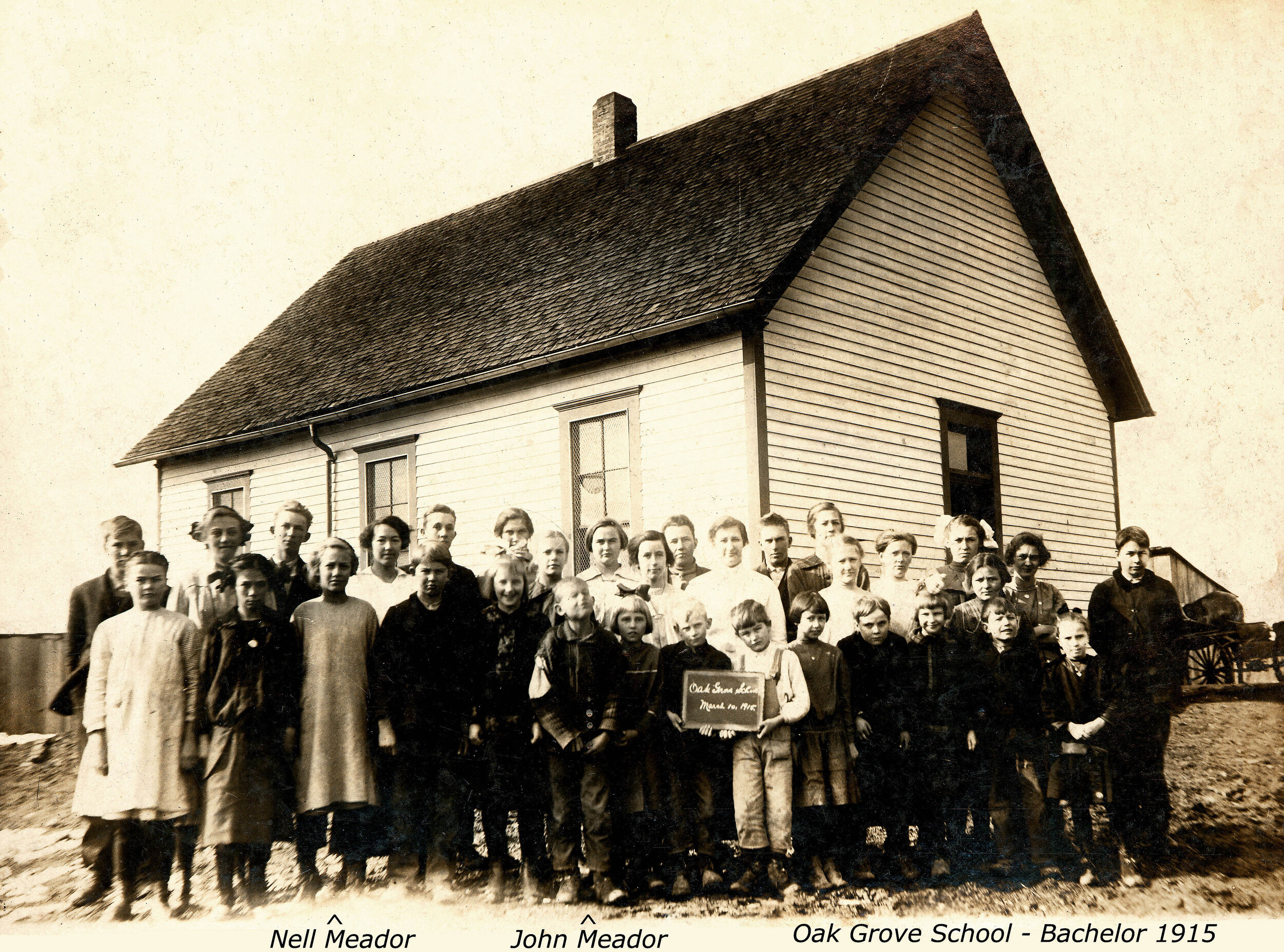This sepia-toned photograph from 1915 captures a group of children and a teacher in front of the Oak Grove School in Bachelor. The bottom of the image contains handwritten labels identifying individuals as Nell Meador and John Meador. The scene features a diverse group of students ranging from young children to older students, all lined up in front of a school building that resembles a house—a common practice for schools at that time. The wooden structure of the schoolhouse includes a door on the right side and three windows. The boys are dressed in long pants and tennis shoes, while the girls are in dresses. A teacher, identifiable by her white blouse with a high neckline, stands slightly off-center to the right among the students. The sky is visible in the background, adding to the nostalgic ambiance of this early 20th-century photograph.